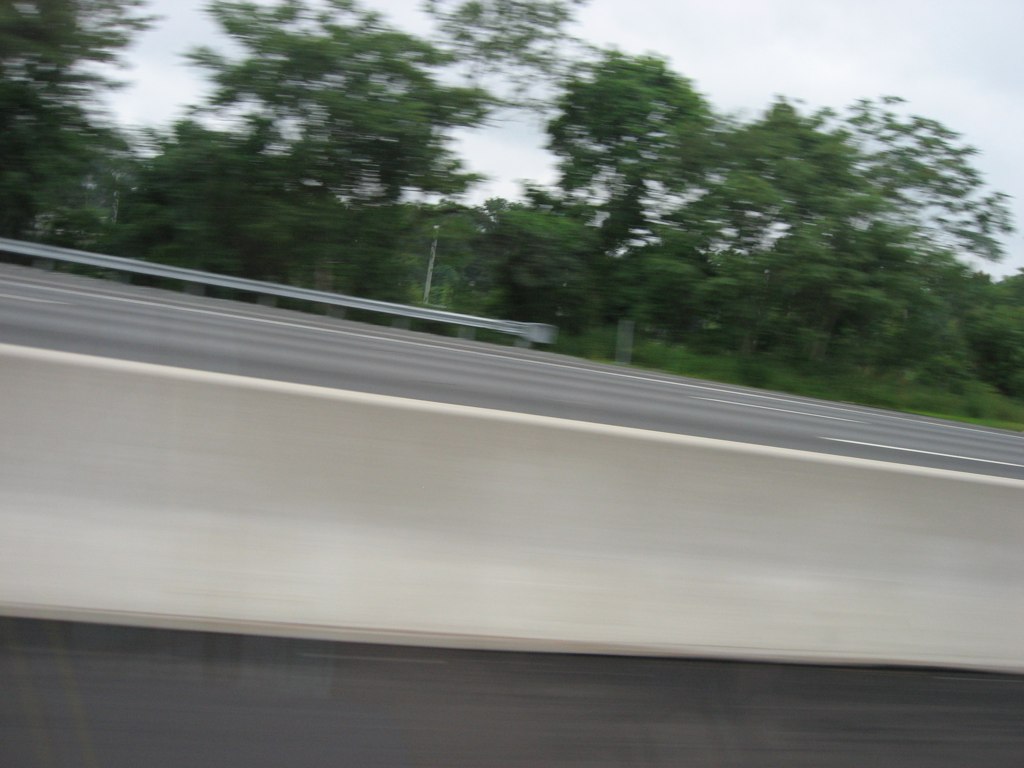A blurry photograph captures a highway scene tilted downwards to the right. The sky is slightly cloudy with numerous green trees lining the background. A highway railing runs from the upper left to the center of the image, merging seamlessly into the asphalt road marked with white lines. Another highway railing can be seen on the opposite side of the road. In the middle section of the photo, a distant telephone pole is faintly visible, while the open, cloudy sky occupies the upper right corner. The lower portion of the image is obscured by a black section, possibly the edge of the camera or a shadow.